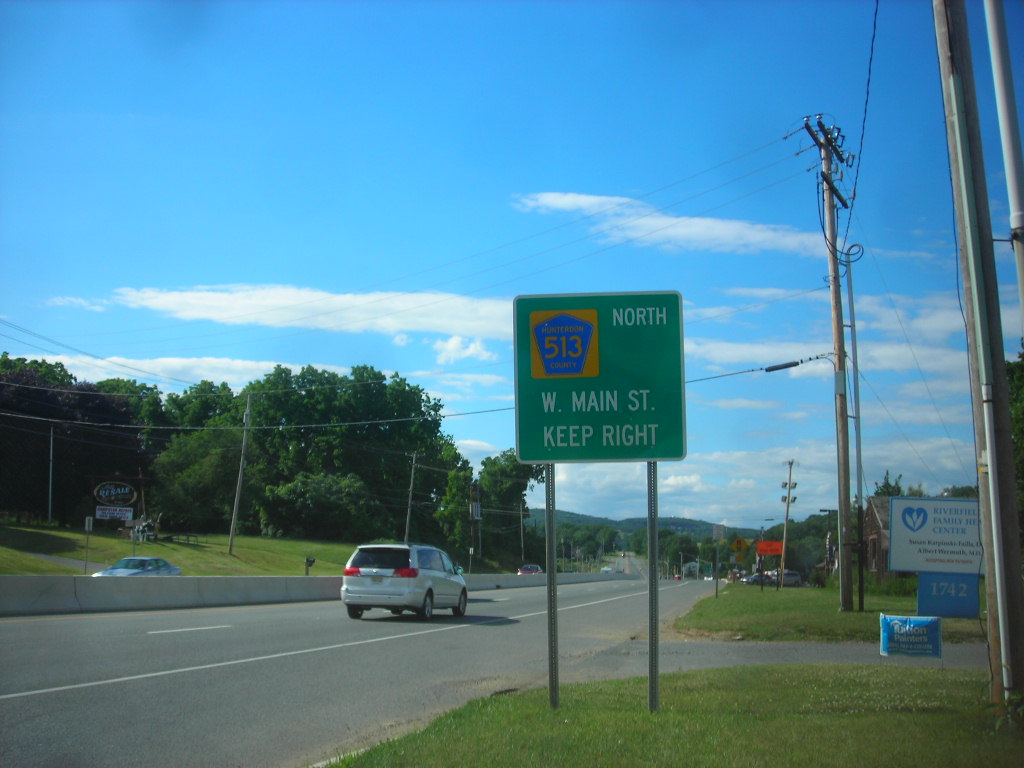This photograph captures a stretch of Highway 513, as viewed from a northbound vehicle. Dominating the lower right corner is a green sign indicating the way to a family health center. The highway itself is divided by a sturdy concrete barricade, separating our three lanes—two for driving and one serving as a drivable shoulder—from the three lanes heading south. Further along, the road descends slightly, emphasizing the downgrade ahead.

To the right, there's an entryway leading to a side parking lot. In the distance, a quaint village is nestled among tree-lined hills, typical of the northeastern United States. A motel occupies the upper left of the image, hinting at roadside hospitality. The sky overhead is a brilliant blue, dotted with puffy clouds, and power lines stretch across the road above, adding an industrial touch to the scene. A light-colored van is visible on the highway, completing this vivid snapshot of American road travel.